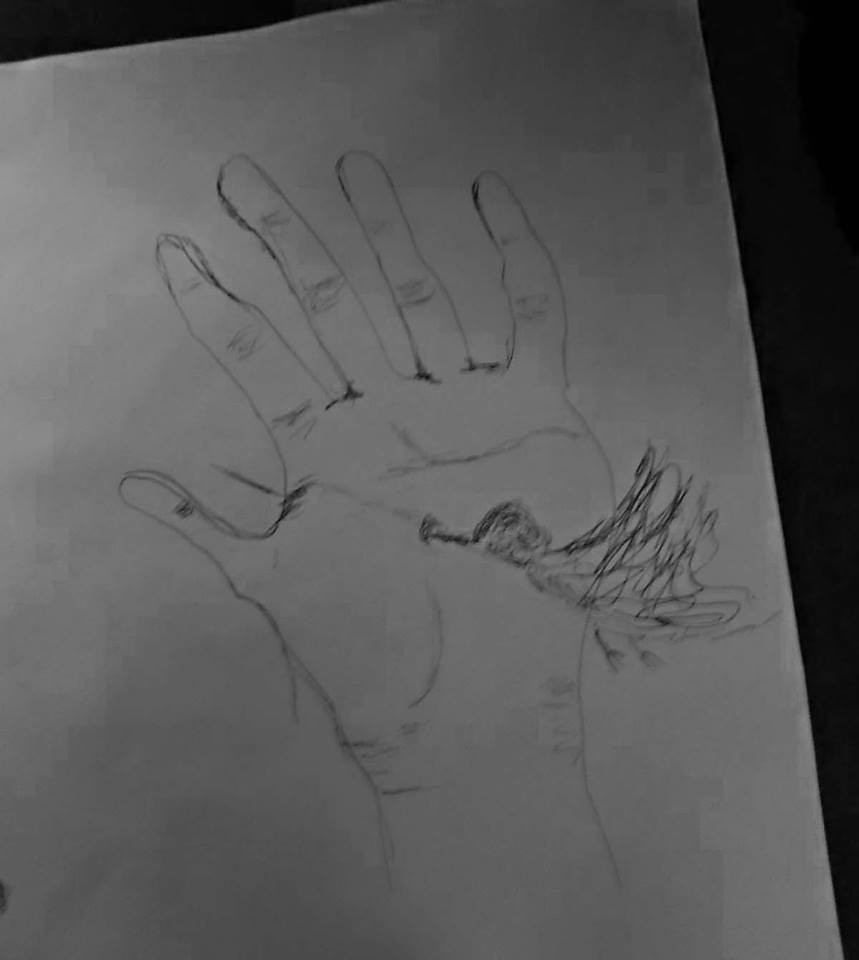This photograph captures a detailed pencil sketch on a white piece of paper, depicting an open human hand with the palm facing up. The hand is illustrated primarily with an outline and a few lines indicating wrinkles. In a dramatic and surreal twist, a scribbly, fluffy hummingbird is shown piercing the center of the palm with its unusually long beak. The bird appears to be flying straight into the hand, with its beak protruding out the backside, just below the thumb and first finger. The hummingbird's form, including wings, tiny feet, and head, is discernible despite the sketchy style, creating a striking and intense visual narrative.